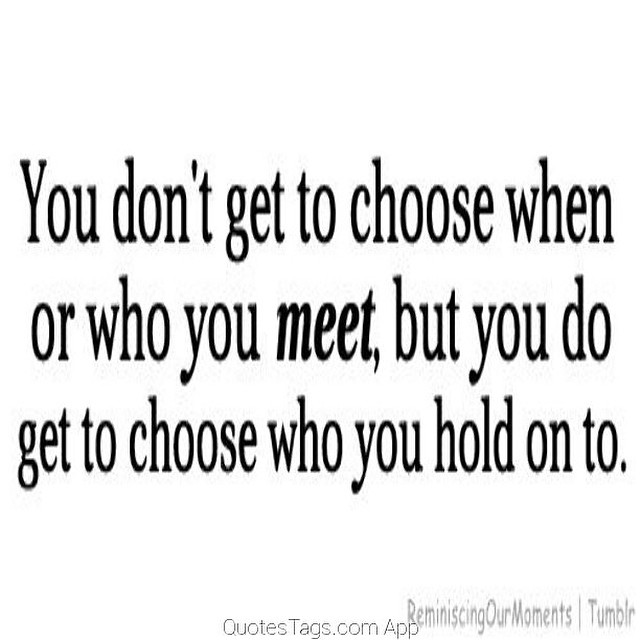The image features an inspirational quote centered on a completely white background, with the text in bold, black font. The quote reads, "You don't get to choose when or who you meet, but you do get to choose who you hold onto." The word "meet" is highlighted in bold. Below the quote, there are footnotes in light gray text, which include "reminiscent our moments / Tumblr" and "quotes tags.com app." This minimalist design emphasizes the text, making the message the focal point of the image.